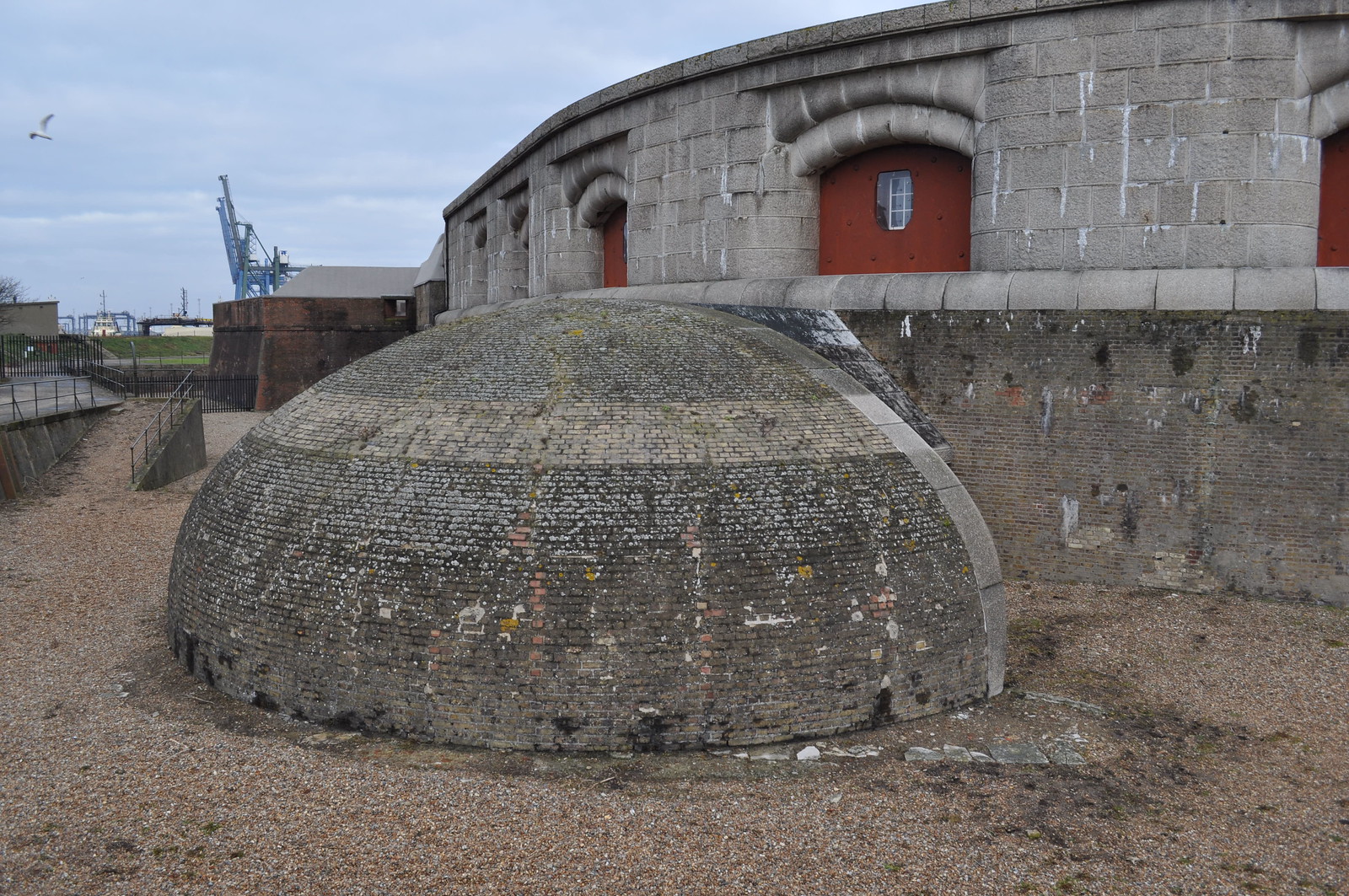The photograph captures an outdoor scene of what appears to be an old, renovated fort or industrial building with a distinct curved, one-floor structure. The lower sidewall of this building features dark brown and dark green colors with black patches, while the upper part is constructed from gray-colored bricks, adorned with several windows encased in red coverings. In front of this main structure, there's a smaller, tomb-like semicircular dome made from dark gray and brown bricks. The sky above is light blue, filled with clouds, and a bird can be seen in the scene. In the background, industrial elements such as a large blue crane are visible, suggesting the location might be near a shipping container loading dock. The area surrounding the building is gravel-covered, further accentuating the industrial yet historical feel of the site.